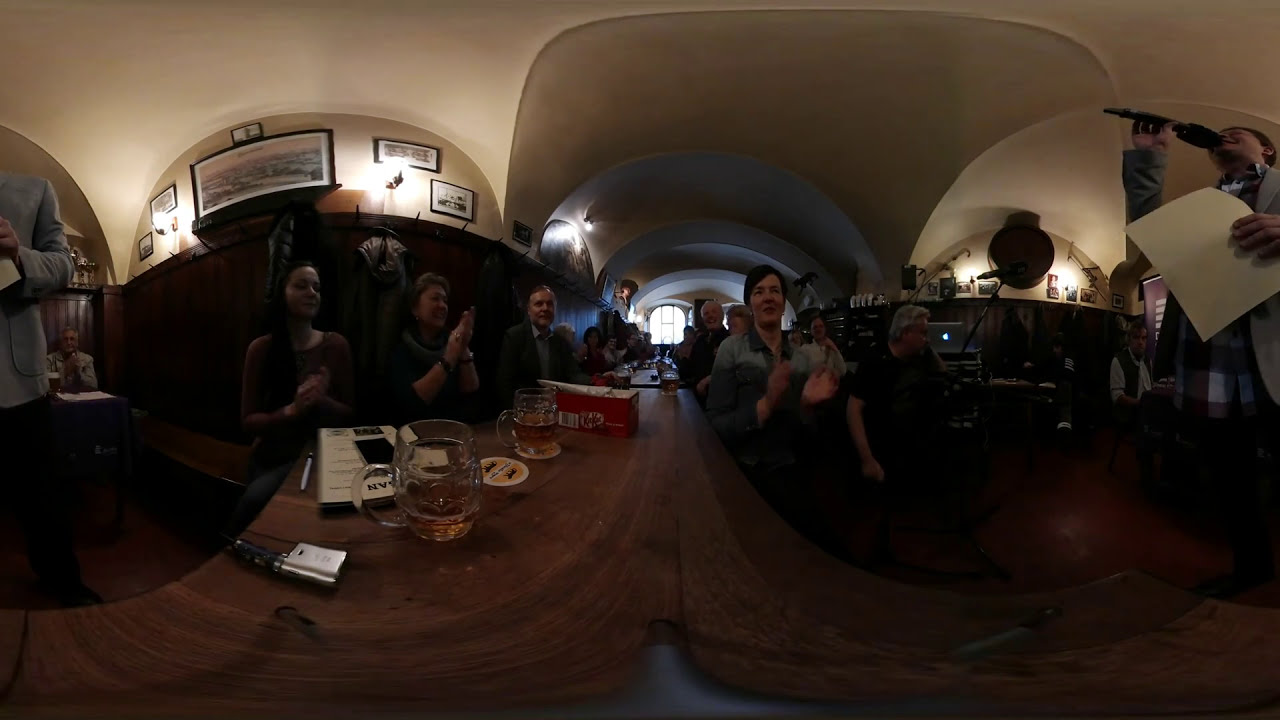The image captures a lively and festive scene set indoors, likely in a bar or restaurant, characterized by a warm, welcoming atmosphere filled with various hues of brown, silver, black, white, red, yellow, orange, and tan. Centered in the photo is a large wooden table, surrounded by several people who appear to be enjoying a celebratory event. On the table are steins of beer and coasters, contributing to the convivial ambiance.

To the right of the image, a person holds a microphone to their mouth, suggestive of a performance or speech, while holding a white piece of paper with their left hand. The backdrop includes numerous paintings or photos in frames hanging on the wall, contributing to the cozy indoor setting. Visible through arches that span the room from left to right are windows that allow natural light to filter in.

In the middle of the image, directly in front of the large table, a gentleman claps enthusiastically, joined by others seated at the table who are also clapping, emphasizing the celebratory nature of the gathering. The counter extends into the background where more people are seen clapping, deeply engaged in the festivity.

To the far left edge, part of a figure stands, dressed in a light blue outfit and dark pants, adding to the layered composition of the setting. In the background, a person with a light-colored jacket or shirt and graying hair is seated with a mug of beer before them, contributing to the bustling yet intimate atmosphere.

All these elements together create a vivid depiction of a joyful moment, with people united in celebration, a performer captivating their attention, and a rich tapestry of visual details that draw the viewer into the scene.